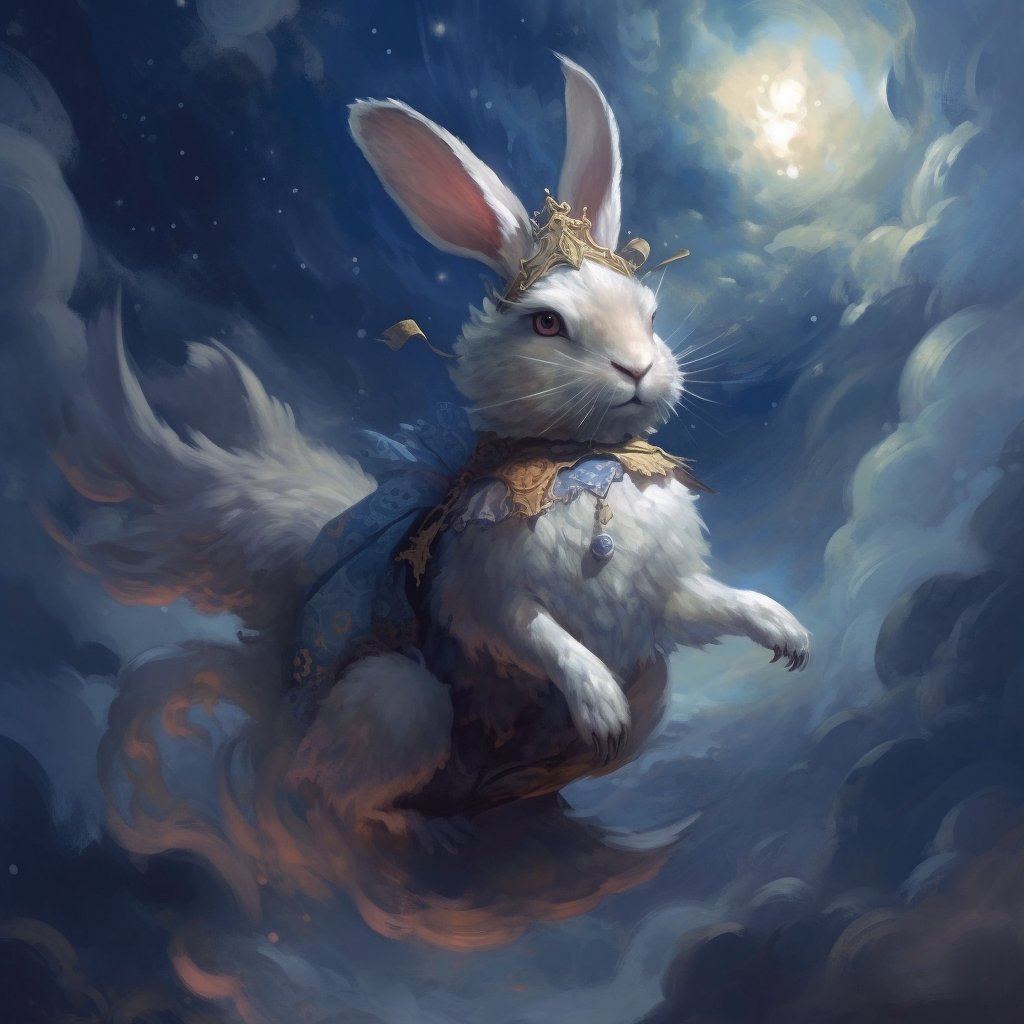In this highly detailed digital painting set within a fantastical dreamscape, a majestic white rabbit soars through a sky tunnel brimming with clouds. The rabbit's ethereal journey takes place against a backdrop where vibrant blue sky melds seamlessly with wisp-like white clouds, hints of covered sunshine, and a sprinkle of twinkling stars. The front paws of the rabbit stretch outward, adorned with sharp, detailed claws, giving it a sense of both grace and strength.

This mystical creature is crowned with a regal, golden crown that fits snugly between its tall, pink-inside ears, which gives it an air of royal distinction. Additional fantastical elements include a blue and cream-colored garment draped around its neck, complemented by a blue pendant necklace. Interestingly, part of the rabbit's form appears to dissolve into wisps of cloud, blending effortlessly into the dreamlike surroundings. The combination of these elements not only highlights the surreal, computer-generated artistry but also imbues the rabbit with an undeniable aura of mythic charm and surreal beauty.